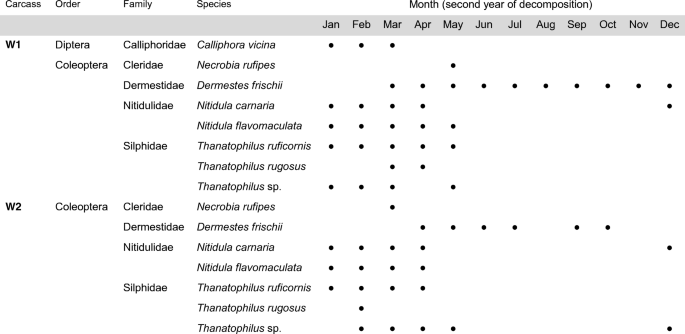The image depicts a detailed, black-and-white scientific chart analyzing decomposition over the second year. The chart is organized into several sections, with the leftmost column listing "Carcass" divided into two segments, W1 and W2. To the right of the carcass column are headings for "Order," "Family," and "Species," each populated with various scientific classifications such as Foridae, Claridae, Dermestidae, and Siphidae. The top of the chart features a timeline spanning from January to December, indicating the months. Throughout the chart, numerous black dots appear under each month within designated rows, indicating occurrences or data points for each species during those months. Notably, the center months (January through April) show a higher concentration of dots, signifying more frequent observations or events. This chart serves as a comprehensive representation of how different species are involved in the decomposition process over time, specifically during the second year.